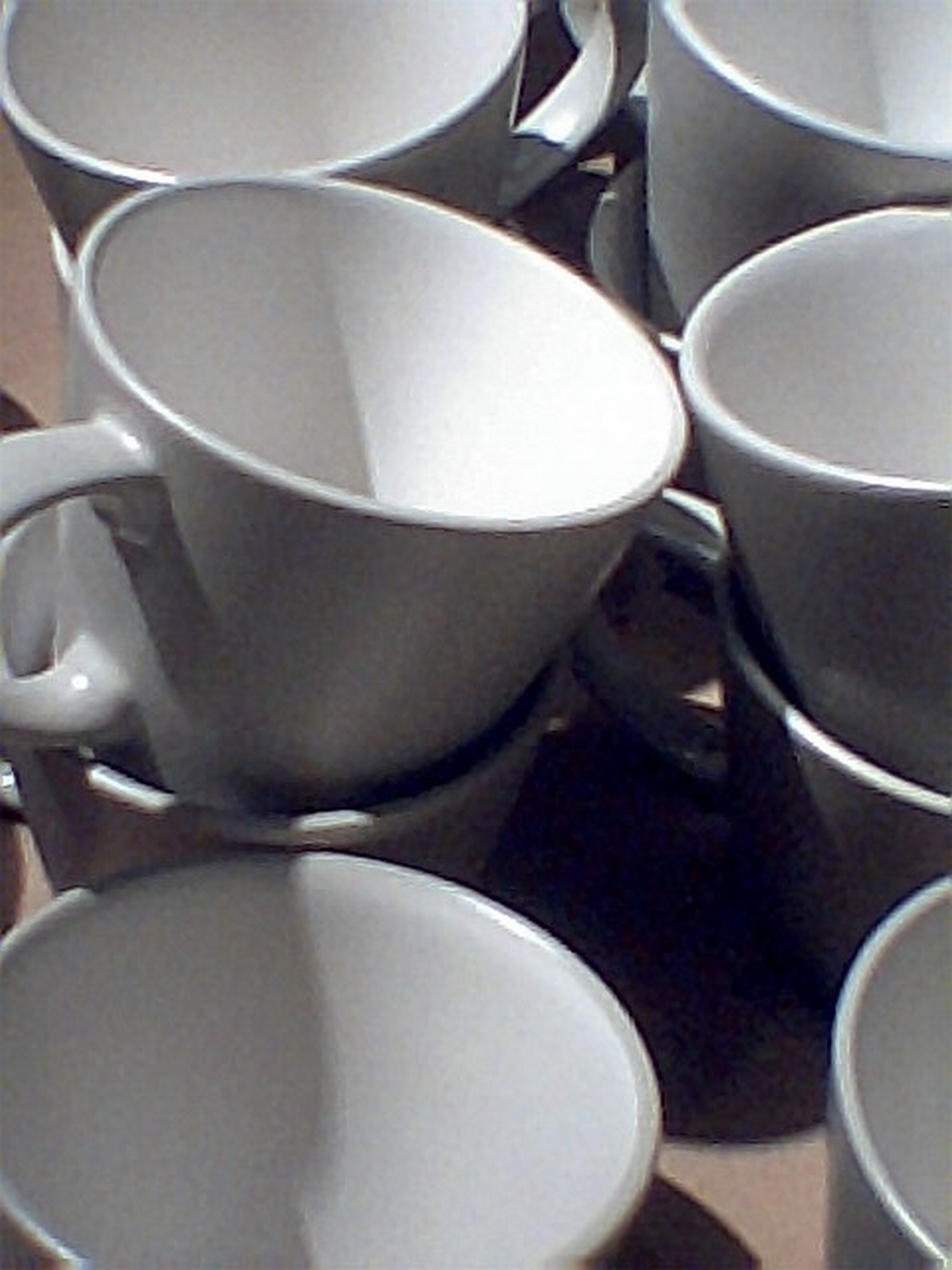The image is a vertical rectangle, showcasing a realistic close-up photograph of ten white ceramic coffee cups, which could also be used for tea. These cups are arranged on a light brown or beige surface, with a dynamic play of lighting and shadows across them. The photo captures varying angles, making some parts of the cups more illuminated while others are in shadow, giving a grayish tint to the exterior. The cups are mostly stacked in pairs; four pairs are arranged one on top of the other, while there are two singular cups positioned at the front. The photo composition is tight, causing many of the cups to be partially cut off. There's no text, logos, or designs on the cups—they are purely white, inside and out, with simple handles. The overall effect is a clean, minimalist presentation that emphasizes the cups' form and the interplay of light and shadow.